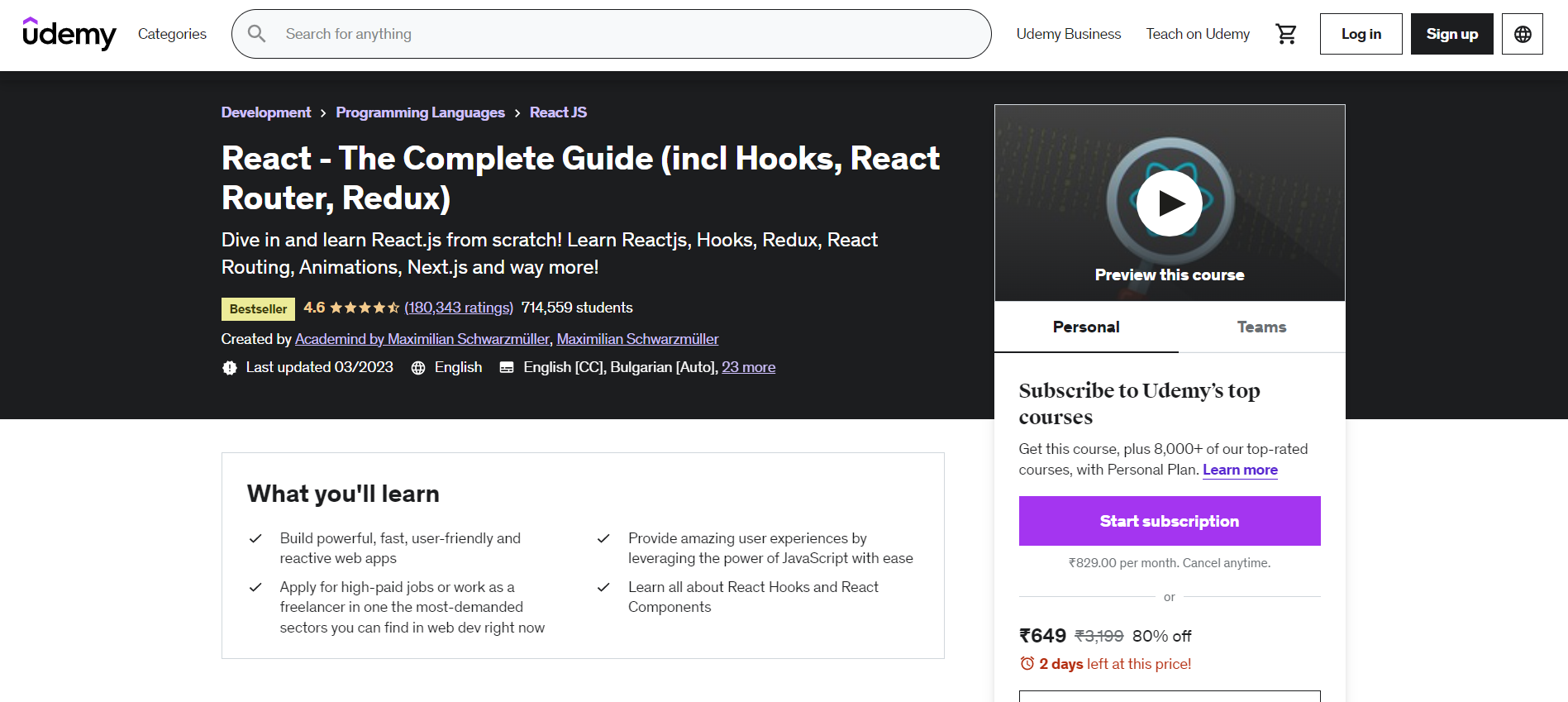Screenshot of Udemy Webpage Detailing Popular Course

The screenshot captures the Udemy homepage, specifically focusing on the navigation bar and a prominent featured course. At the top of the image, there is the "Categories" section, followed by a search bar. Positioned to the right of the search bar, the options include "Udemy Business," "Teach on Udemy," and icons for a shopping cart, "Log In," and "Sign Up."

A black banner below the navigation bar highlights various course categories such as "Development," "Programming Languages," and "React.js." The featured course is titled "React - The Complete Guide (incl Hooks, React Router, Redux)" and promises comprehensive instruction on React.js, hooks, Redux, React routing, animations, and Next.js along with additional topics.

Details of the course emphasize its popularity and credibility:
- Best Seller designation
- 4.6 out of 5 stars based on 180,343 ratings
- 714,559 enrolled students
- Created and instructed by Maximilian Schwarzmüller
- Last updated in March 2023
- Offered in English with English closed captions and Bulgarian auto captions, along with 23 other languages

Additional offerings include a course preview and options for personal and team subscriptions. The personal plan provides access to this course and over 8,000 top-rated courses on Udemy for a monthly fee of $29.99 with the flexibility to cancel any time.

Currently, the course is available at a discounted price of $64.99, marked down from $319.99, offering 80% off for the next two days.

Key Learning Outcomes include:
- Building powerful, fast, user-friendly, and reactive web apps
- Gaining skills to apply for high-paying jobs or work as a freelancer in the web development sector
- Providing outstanding user experiences by effectively leveraging the power of JavaScript
- Mastering React hooks and React components